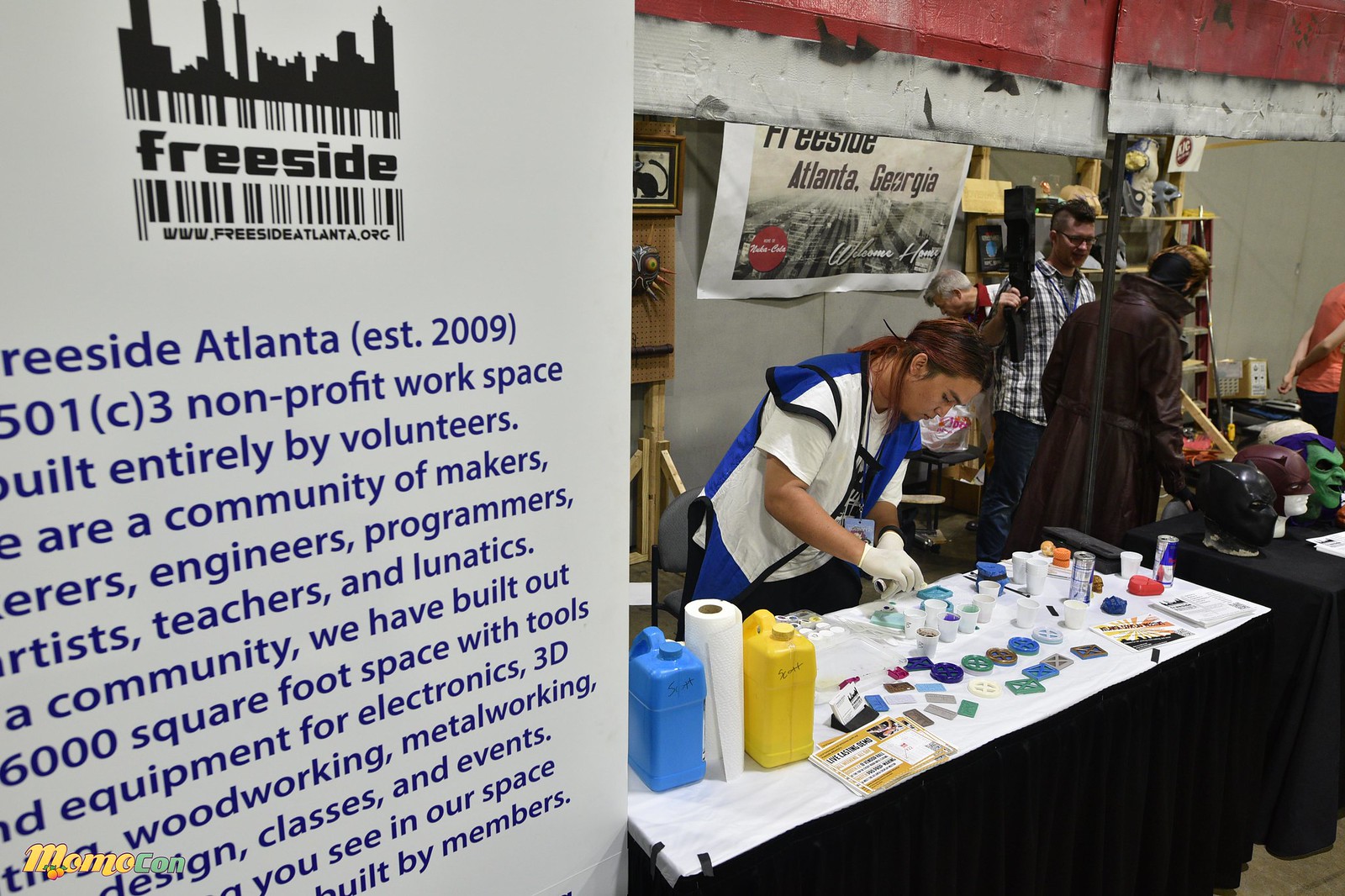The image depicts a bustling indoor festival or event, prominently featuring the vibrant community organization, Freeside Atlanta. To the left, there is a large white board adorned with a logo that reads "Mall Me Calm. Freeside. Freeside, Atlanta. Established 2009," detailing that Freeside is a 501c3 nonprofit workspace entirely built by volunteers. The sign on the board highlights their extensive 6,000 square foot space equipped with tools for electronics, 3D printing, woodworking, metalworking, and design, and emphasizes their community made up of makers, engineers, programmers, artists, teachers, and enthusiastic creatives. Visitors can observe the diverse activities facilitated in this space. 

On the right side of the photo, a table is set up with a black skirt, where an Asian woman wearing white gloves is engrossed in a craft project involving small Dixie cups filled with various liquids, presumably paints. The environment is enriched with artistic hustle, as seen with a man working on an art project nearby and people in the background engaged in creating superhero masks, such as those resembling Black Panther, Daredevil, and Green Goblin. Behind them, a banner emblazoned with "Freeside, Atlanta, Georgia" affirms the strong community spirit and creative energy that permeates the space. Decorations on the walls add to the festive and collaborative atmosphere of the event.